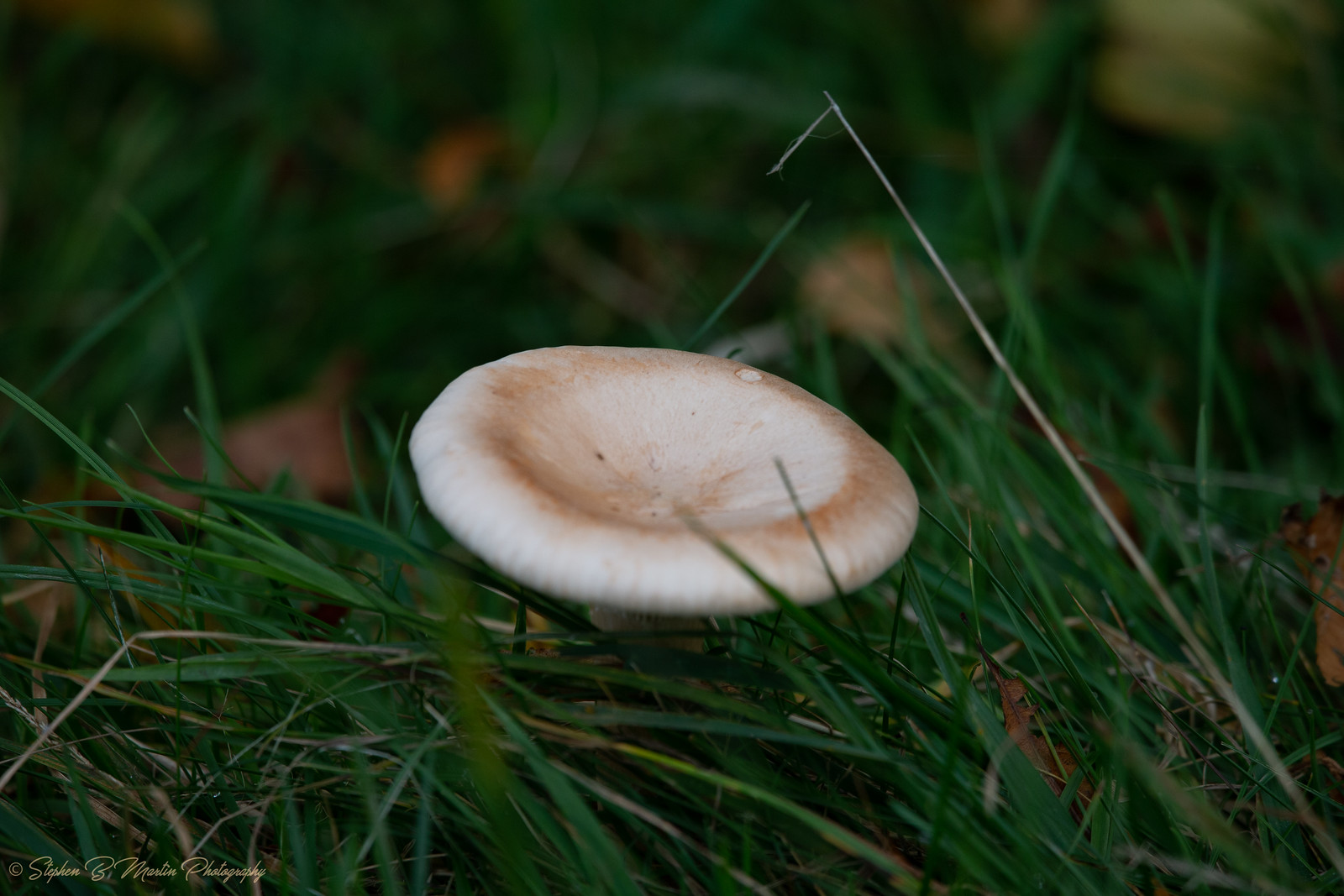This is a close-up photo of a distinctive mushroom growing in a lush, green grassy area. The mushroom has a flat, circular cap with a noticeable dip in its center, and exhibits a white coloring with subtle pink and orange tones, particularly around its rim where the shade deepens to a darker orange. It is relatively short, as evidenced by the grass, which, although some blades have been pushed down, still appear about twice the height of the mushroom. The background fades into a blur, hinting at additional mushrooms and tall grass, but keeping the focus firmly on the foreground. The grass, healthy and vibrant, fills the scene with occasional brown leaves interspersed. In the bottom left corner of the image, there is cursive gold text for copyright, legibly stating "Stephen B. Martin Photography."